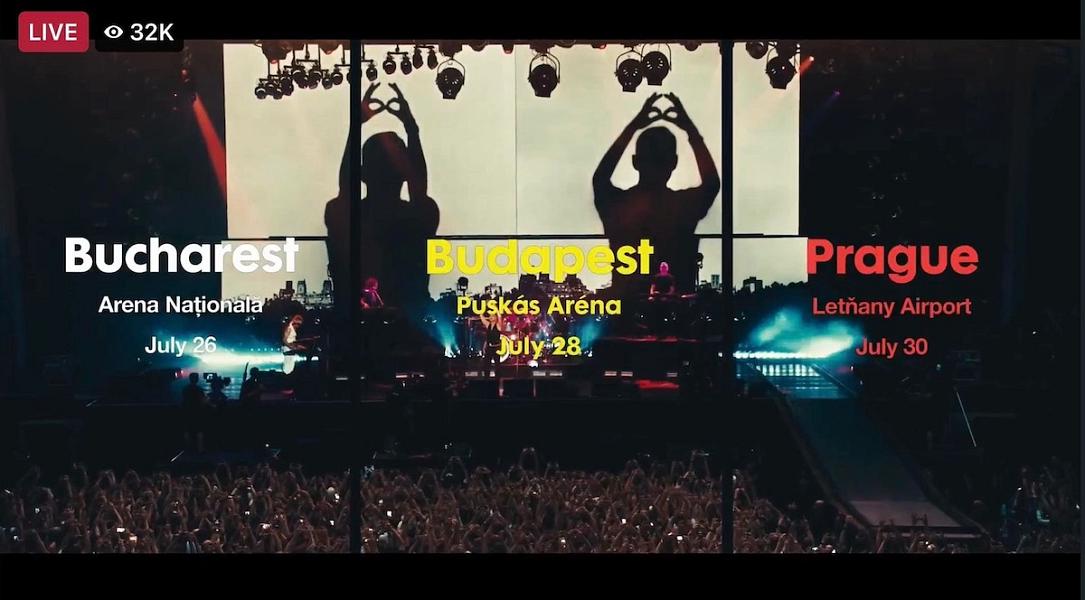This image appears to be a promotional graphic for a live concert tour, possibly streamed on YouTube. In the upper left corner, there is a red "LIVE" button with white text, and next to it, an eye icon accompanied by the number "32k" in black, indicating viewership. The image consists of three sections, each showing large crowds at a concert, with fans raising their hands in unison to create a "goggle eyes" gesture, reflecting a shared concert tradition. Each section is divided by thin bars, containing information about different concert dates and locations:

1. The left panel, with white text, reads "Bucharest, Arena Națională, July 26th."
2. The middle panel, in yellow text, states "Budapest, Puskás Aréna, July 28th."
3. The right panel, with orange text, details "Prague, Letňany Airport, July 30th."

On stage, a large screen silhouettes performers, who are orchestrating the crowd's movements. Hundreds of smartphone lights are visible among the audience, capturing and recording the event. The stage is predominantly dark, illuminated by blue lights emanating from various points behind the band, creating a dramatic and engaging atmosphere. The image emphasizes the strong and enthusiastic fanbase of the band, whose identity remains unspecified in the description.